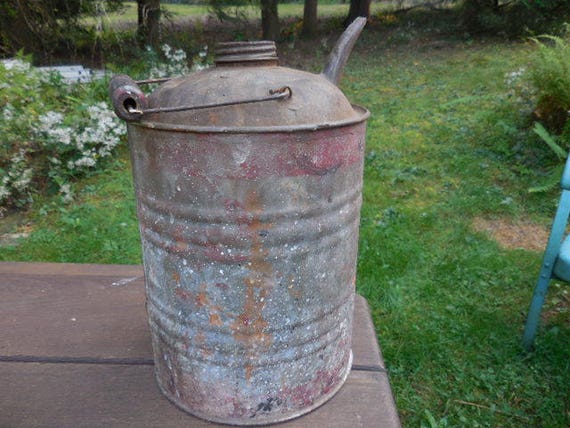This image depicts an old, rusted kerosene gas can, approximately one foot tall, notable for its weathered and well-used appearance with paint splatters, especially around the bottom, and extensive rust in varying hues of red, orange, and turquoise. The can features a rounded top with a spout jutting out from the side and a wooden handle lying down on the left. It sits on a wooden platform, possibly a picnic table, positioned in the lower left-hand corner of the image. The photo is taken outdoors in a backyard garden, with lush green grass visible in the background. To the left, there are white flowers on green stems and a bush, while a few trees stand further back. A partial view of a leg from a blue chair can be seen in the mid-right area of the frame, contributing to the rustic garden setting.